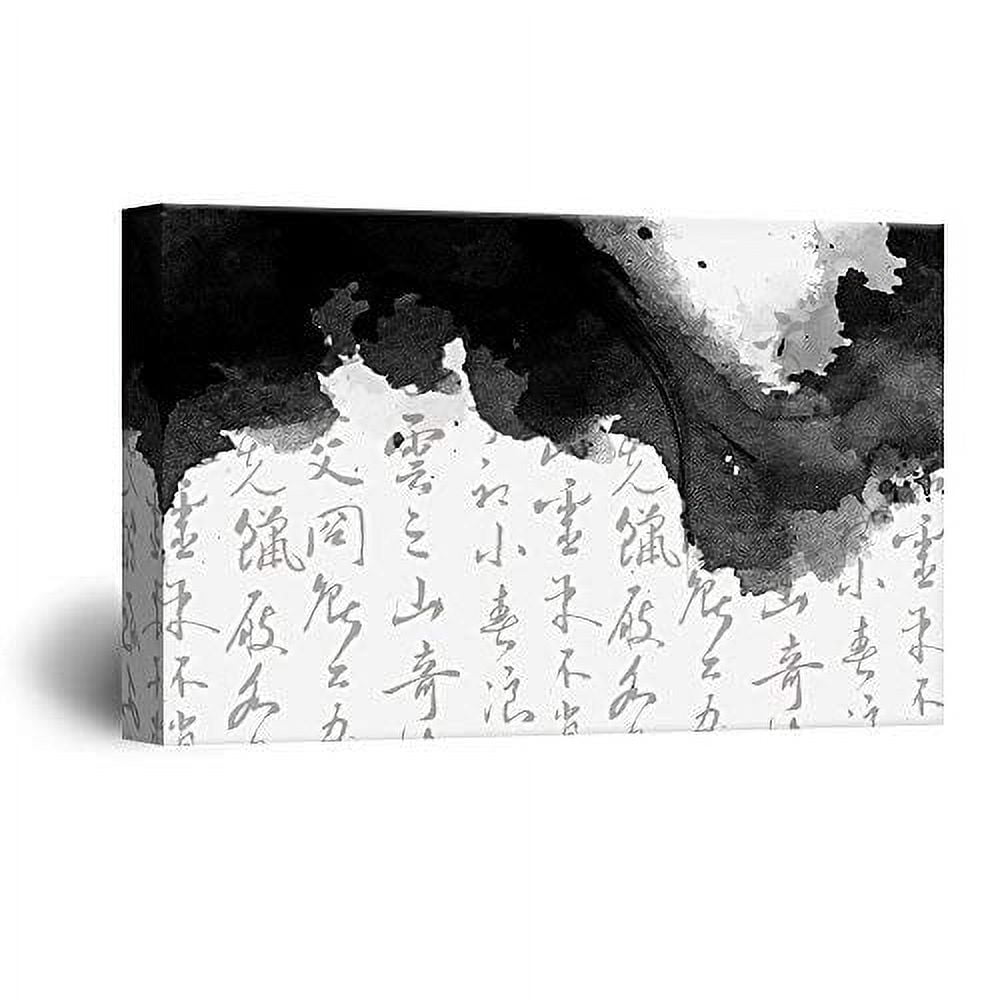This black and white image features a narrow, worn cardboard box standing upright. The box, originally white, prominently displays Oriental-style text, likely Chinese characters, across its entire visible surface. Positioned on a stark white background, the box casts a distinct shadow to the bottom left. The box is noticeably deteriorated; the wear and tear have exposed darker materials beneath the surface, creating a patchwork of black and grey shades where the text has faded away. The image captures the worn textures and contrasts that tell the story of the box's age and fragility.